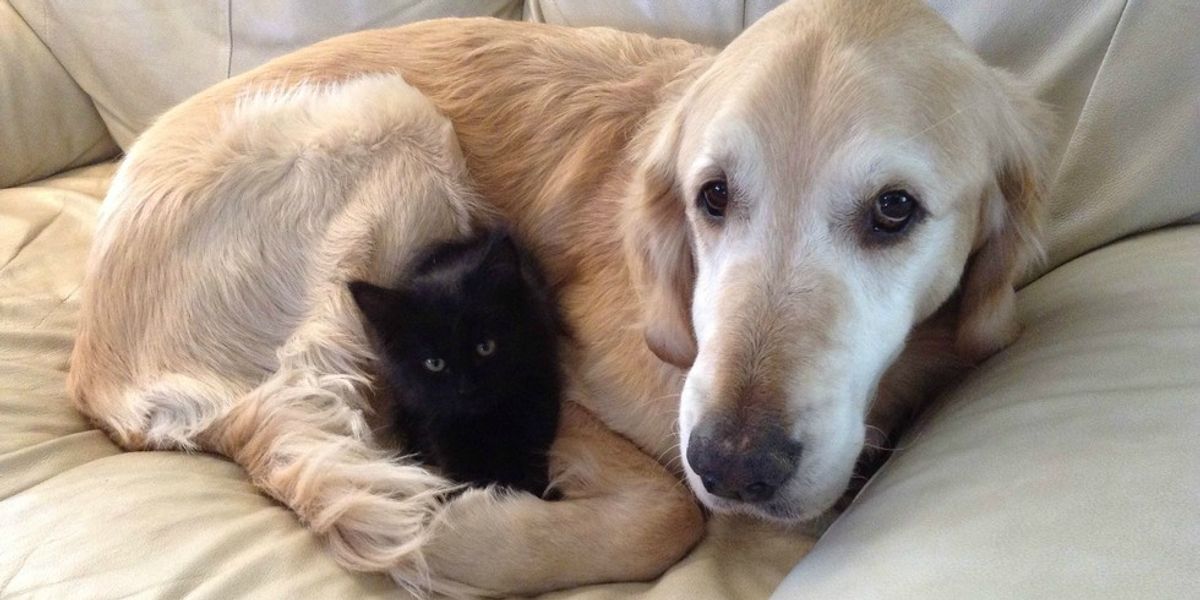In the center of the image, a brown and white dog is resting, curled up comfortably on a light beige, padded couch that appears to be made of a suede-like material. The dog's head, which features light brown fur with white markings around its eyes, is turned slightly to the left, showing its droopy ears and sad, dark eyes. Its snout is long, with a black nose, and its body's lighter brown and white fur is visible from its back and torso. Nestled snugly between the dog's front paws and back legs is a small black kitten, only its head, a bit of its back, and its striking green eyes clearly visible. The image is framed by the light-colored couch, with a cushioned armrest appearing to the right of the dog's head and the backrest of the couch stretching behind them, adding to the scene's cozy ambiance.